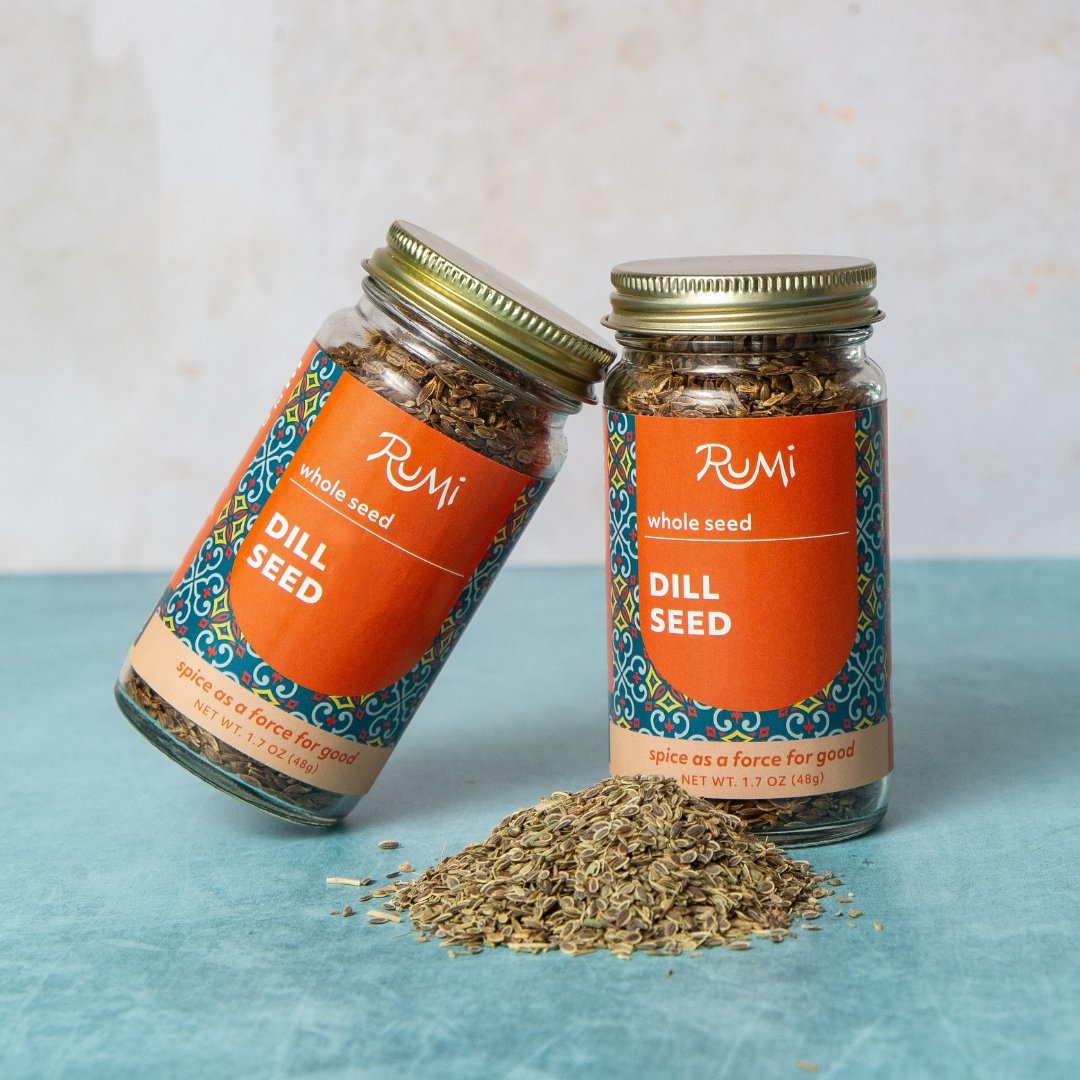This detailed image showcases two jars of dill seed prominently displayed on a blue countertop with a plain white background. Both jars have gold lids and are adorned with vibrant orange labels featuring intricate blue, yellow, and red designs. The labels read "Rumi, whole seed, dill seed," with an additional creamy beige label at the bottom in orange font stating, "spice as a force for good." The jars are similarly labeled and weigh 1.7 ounces (48 grams) each. One jar is positioned upright, while the other leans against it at an angle. In front of these jars, a small heap of dill seed is scattered on the countertop, enhancing the visual appeal of the spices. Both jars appear densely packed, emphasizing the richness of the product within.